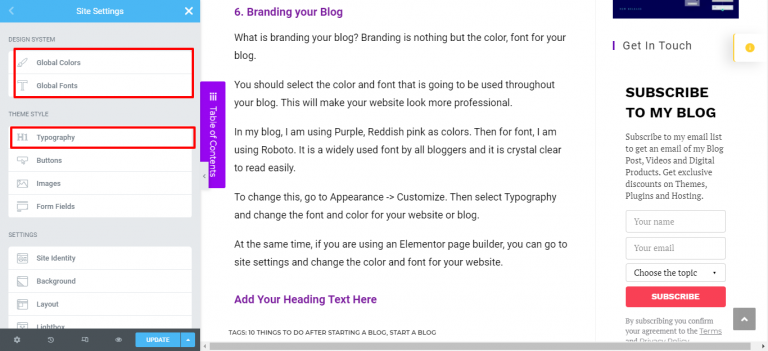In the provided image, we are examining a detailed screenshot of a website's settings page. At the top-left corner, there's a blue rectangular background labeled "Site Settings." Directly beneath this section, you will find a light gray background filled with white rectangular rows containing various options. The first row features two options: "Global Colors" and "Global Fonts," highlighted by a red rectangle. Below this, additional rows include options such as "Theme Style," with sub-options like "Typography," "Buttons," "Images," and "Form Fields." Following that is the "Settings" section, which lists "Site Identity," "Background," "Layout," and other options, though some are obscured at the bottom.

On the right side of the image, the phrase "Branding your Blog" is prominently displayed in purple text, accompanied by several sentences in black text elaborating on the topic. Further down, the section prompts the user with "Add your Heading Text Here" in purple, adjacent to a dark blue rectangle at the top.

Below this, there's a section inviting user interaction, beginning with "Get in Touch." This area features a white square with a yellow circle in the center and a small yellow line along the left edge of the square. Beneath this are instructions for subscribing to the blog, rendered in black text: "Subscribe to My Blog," followed by a few explanatory sentences. This section provides fields for entering one's name, email, selecting a topic, and concludes with a red "Subscribe" button. Completing the image's layout, a gray bar spans the very bottom of the screenshot.